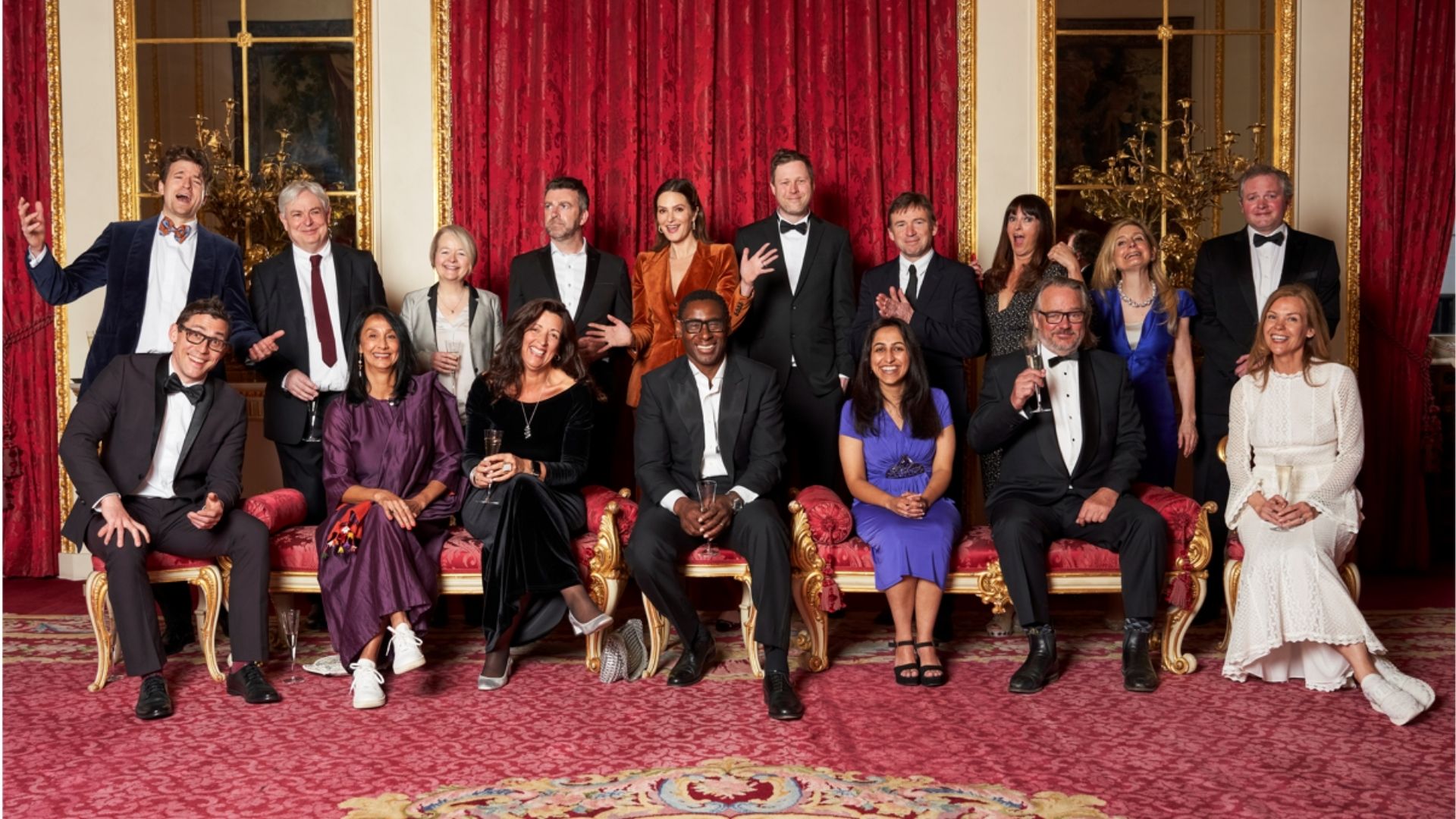A group of well-dressed individuals is posing for a formal photograph. The group is arranged in two rows; the front row is seated on a luxurious bench and chairs, upholstered in rich red velvet with a gold frame. Behind them, the second row is standing. The men are mostly wearing black suits accessorized with bow ties, while the women are in various elegant dresses. Some of the people in the image are holding drinks, adding a casual touch to the otherwise formal setting. The floor is covered with a plush red carpet, featuring an intricate yellow design in the center. The atmosphere exudes sophistication and style, highlighting the group's polished appearance.